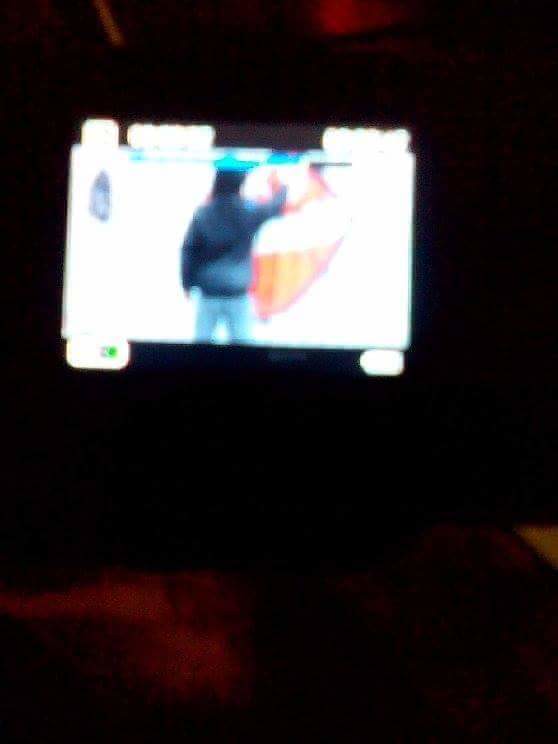Against a predominantly dark backdrop, shades of black and deep purplish-pink dominate the scene, creating a striking contrast. The central focus of the image appears to be a brightly illuminated screen, resembling a smartphone that is oriented sideways. The screen displays what seems to be a video game or a digital animation. Dominating the digital screen is an animated character wearing a dark blue coat, with their arm confidently raised in the air. The character is depicted with black hair and is dressed in blue jeans. Adding a vibrant splash of color, a flowing cloth in vivid hues of red, orange, yellow, and pink descends gracefully. The top edge of the screen is punctuated by small boxes that likely represent game icons or interface elements, adding further detail to the lively and dynamic scene.